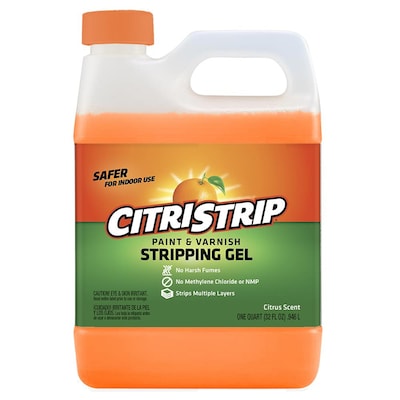This detailed photograph showcases a Citrus Strip Paint and Varnish Stripping Gel, designed for safer indoor use. The gel comes in a clear, white plastic bottle that is roughly one gallon in size, and it is filled with an orange liquid up to about 80% of its capacity. The bottle features an orange plastic cap and a convenient handle located at the top for easy carrying. The label, which wraps around the front and sides, is vibrant with orange, red, and green hues. Central to the label is an illustration of an orange fruit with green leaves, framed with sun-like rays emitting from behind, giving the appearance of a sunburst. The label prominently displays the product name "Citra Strip" in white text, followed by a description stating it is a paint and varnish stripping gel and highlighting that it is safer for indoor use, with the additional note that it has a citrus scent. The entire setup pops against the simple white background of the computer screen, making the colorful elements stand out.